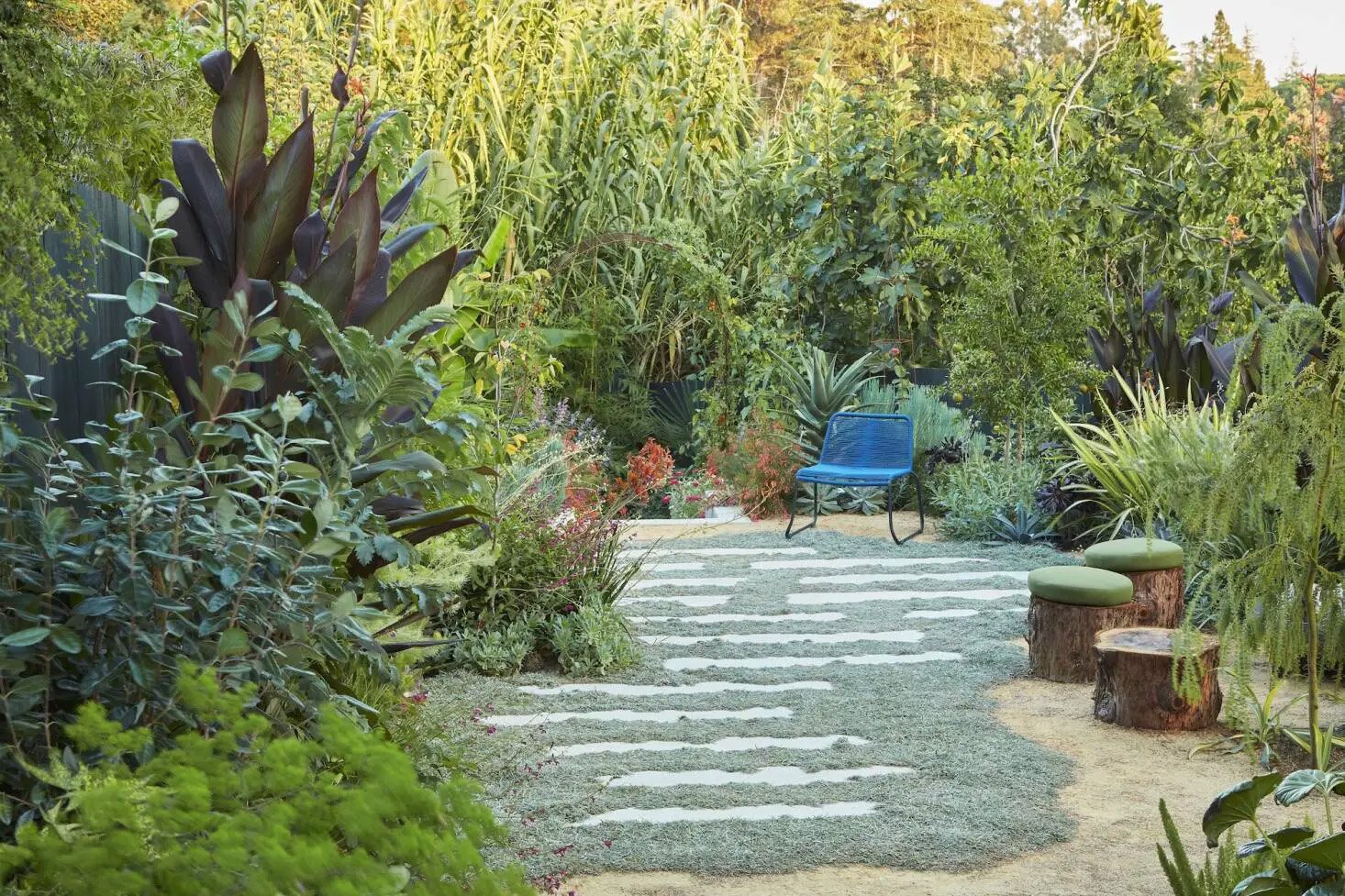The photograph is a horizontal, rectangular image of what appears to be someone's backyard, taken during the day. The majority of the image is filled with an array of lush plants and vegetation, including tall trees and various bushes and flowering plants in a variety of green shades. A pathway made of large white stepping stones intersects the area, laid over a surface that looks like artificial teal-colored turf or grass. 

At the top of the pathway, centrally placed, is a blue outdoor chair with a black metal frame. To the right of the chair are three tree trunk stools, two of which are topped with green pads, while the third is missing its cushion. The ground in this area appears to be bare dirt. The overall setting presents a serene, natural landscape with a combination of meticulously arranged planted areas and informal seating options, inviting relaxation amidst the greenery.